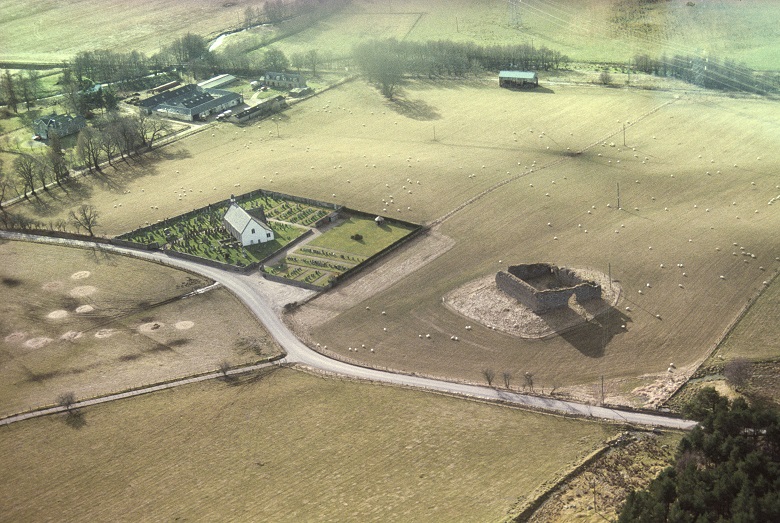This image is an aerial view of a rural scene, dominated by farmland that has been plowed and prepared for planting. The expansive fields primarily appear barren and yellowish-brown, indicating a need for more water. Central to the scene is a white house surrounded by lush, green land, enclosed by a square fence. Near this house is a large container situated on a small bed of dirt. The greenery around the house contrasts sharply with the otherwise dry environment. In the upper left corner, there are additional buildings that are unidentified, surrounded by tree lines and a road. There's another building in the upper center and another road intersecting the scene in the lower right and extending out to the left. In the background, power lines and additional houses are visible, blending into the rural landscape characterized by sparse trees, numerous roads, and extensive farmland.